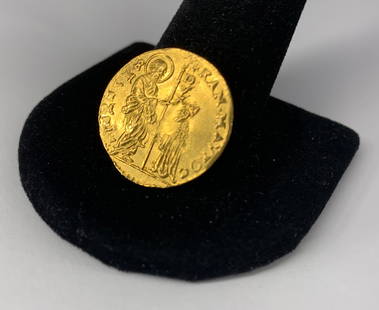In this detailed photograph, we see an artifact that appears to be an ancient coin, roughly the size of an American half dollar. The coin, with a rich gold color, is displayed slightly upright on a black felt-covered stand, set against a plain white background. The coin's surface is shiny, indicating it has been well-maintained, though it shows subtle signs of age with some parts looking slightly dull. The central design depicts two figures: the larger one on the right is adorned with a halo, flowing robes, and is holding a staff or tall stick; the smaller figure on the left, also in robes, seems to be bowing or positioned lower in some respect, and wears a peaked cap. Surrounding this scene is an inscription along the edge, rendered in a foreign language that is hard to decipher due to blurriness.